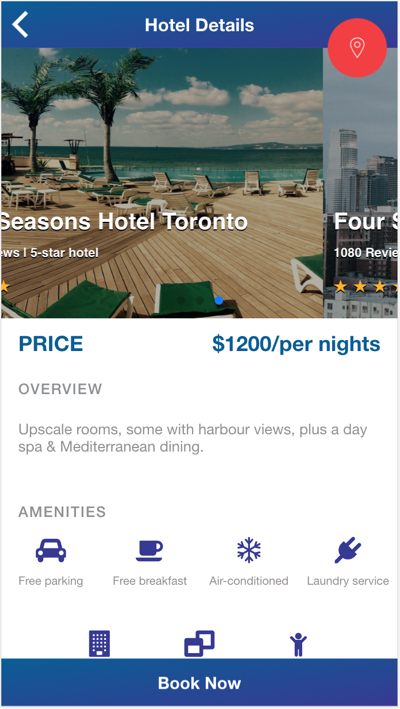This detailed caption describes an image of a mobile screenshot related to hotel booking information:

"The screenshot, shaped like a mobile screen, features a blue header with white text that reads 'Hotel Details,' accompanied by a back arrow in the upper left corner and a red circle with a Google Maps pin symbol in the middle-right of the header. Below the header is a graphic showcasing the name 'Seasons Hotel Toronto WSI,' labeled as a five-star hotel. The image includes a photograph of a long wooden deck furnished with lawn chairs, flanked by two palm trees and overlooking a green-tinted ocean. To the right of this photograph, a partially visible image of a city's skyline is shown, along with the text indicating '1080 reviews.' Below the visuals, the text 'Price: $1200 per night' is displayed, followed by an overview highlighting the hotel's features: upscale rooms (some offering harbor views), a day spa, and Mediterranean dining options. The amenities listed include free parking, free breakfast, air conditioning, laundry service, and three additional icons that are not visible due to the content not being fully scrolled. At the bottom of the screen, a prominent blue button reads 'Book Now.'"